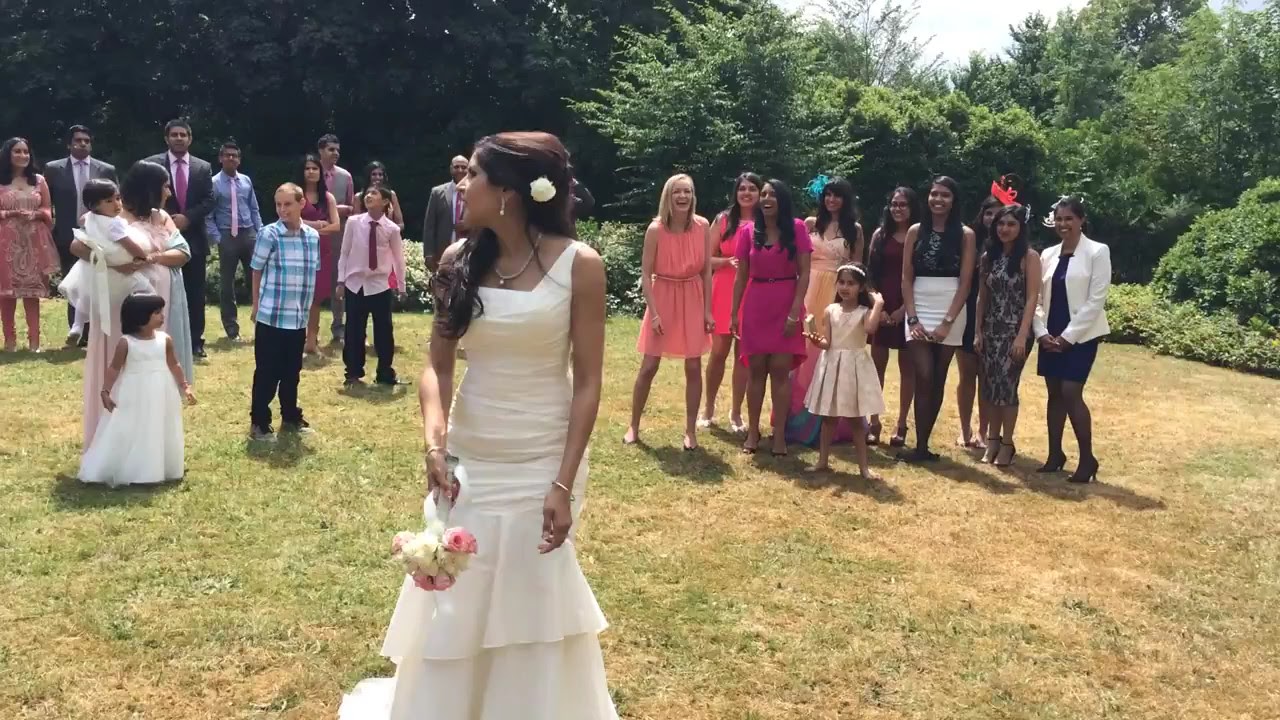In this horizontally aligned rectangular image taken during an outdoor wedding, we see a radiant bride about to throw her bouquet. She stands on a grassy lawn, framed by a backdrop of lush green trees and a partly cloudy sky peeking through the upper right corner. The bride, with long black hair adorned with a white flower and pulled over her right shoulder, exudes elegance in a sleeveless, two-tiered, ruffled white mermaid gown. Her dress features a ruched bodice that accentuates her figure. She faces the camera, with her head tilted to the right, holding a bouquet poised for the traditional toss. Behind her, a group of nine women and a little girl eagerly anticipate catching the bouquet. The women are formally dressed and exude happiness, laughing and smiling. To the left, there are mixed families, including another woman holding a baby in a white dress and a little girl who resembles the bride. The scene is bathed in sunlight, highlighting the joyous ambiance of this special occasion.